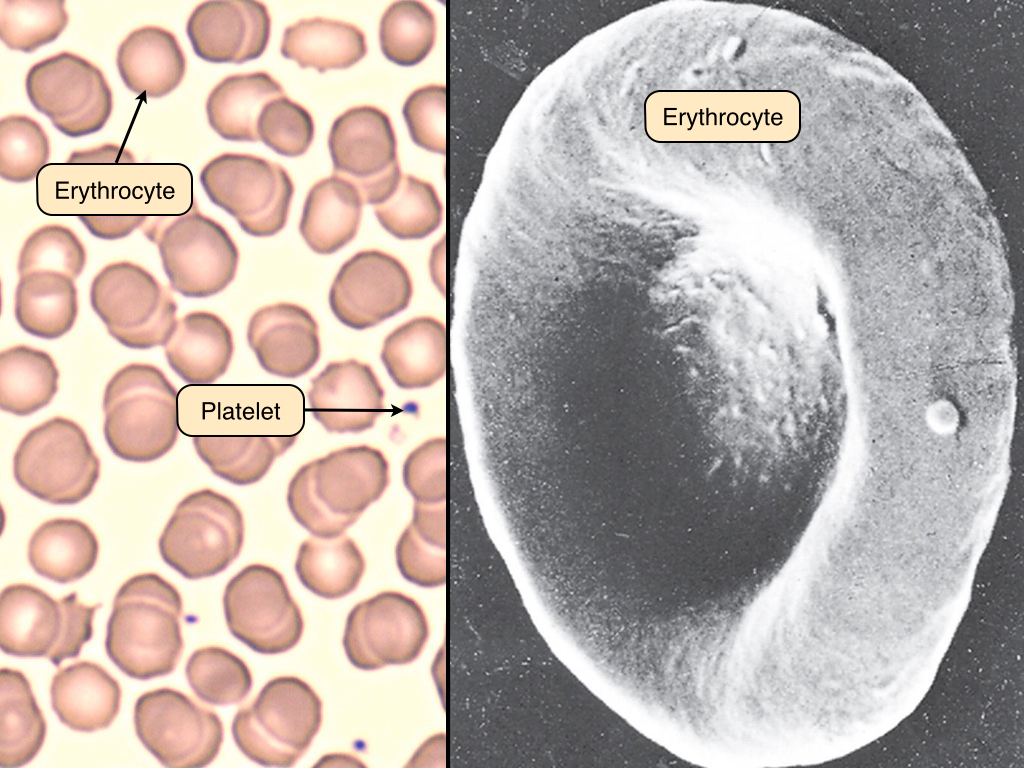The image is a split diagram, often seen in science textbooks, illustrating blood cells. The left side features a light yellow background populated with numerous mauve to maroon, round to oval red blood cells (erythrocytes) and a few purplish platelets. Annotations are provided with yellow boxes bordered in black: one highlights an erythrocyte, and another points to a platelet. The right side of the image presents a highly magnified, black-and-white depiction of a single erythrocyte, prominently showcasing its characteristic donut-like shape with a central indentation. The same yellow box with black text labels this enlarged erythrocyte for clarity.